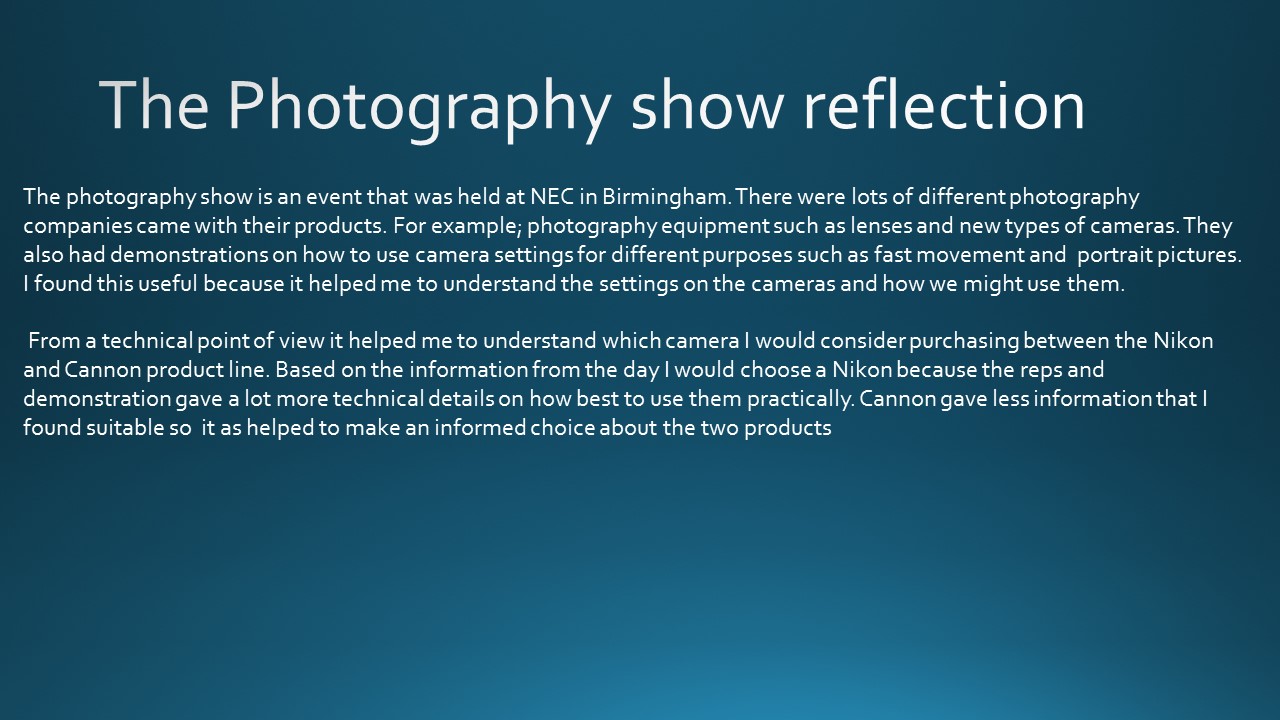The image is a color presentation slide with white text on a medium blue background. The title, "The Photography Show Reflection," is prominently displayed in white, capitalized text at the top. Below the title, two paragraphs of text provide detailed insights into the event. The first paragraph describes The Photography Show, which was held at the NEC in Birmingham and featured a variety of photography companies showcasing their products. This included photography equipment such as lenses and new camera types, along with demonstrations on using camera settings for different photography styles, including fast movement and portrait pictures. The text explains that these demonstrations were particularly useful for understanding camera settings and their practical applications. The second paragraph focuses on the writer's personal takeaways from a technical standpoint. It details the comparison between Nikon and Canon cameras, with the writer favoring Nikon due to the more comprehensive technical information provided by the representatives and demonstrations. This thorough explanation helped the writer make an informed choice, contrasting it with the less detailed information available from Canon.